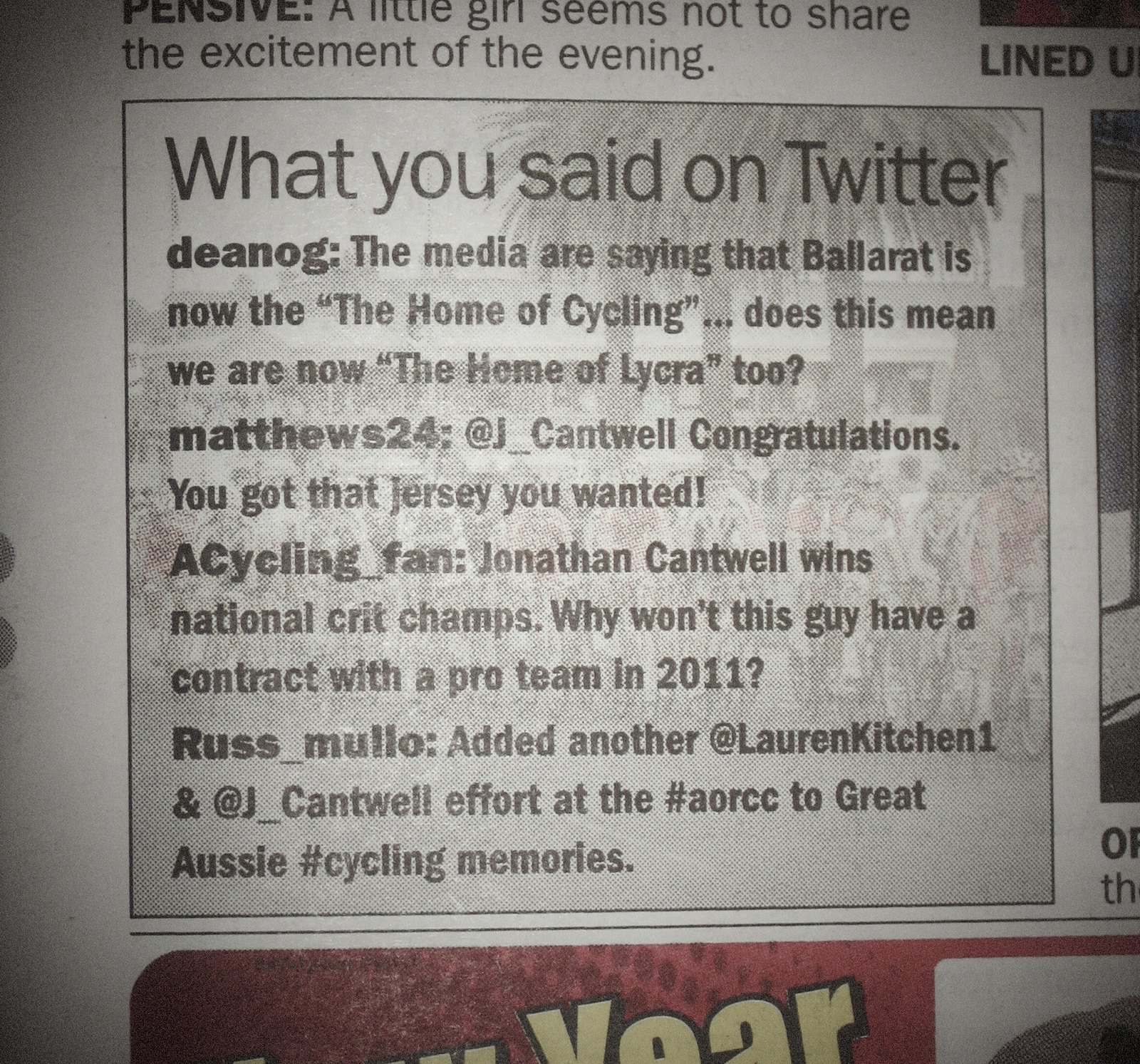This is a section from a newspaper or magazine featuring a visually dynamic layout centered around cycling. The main element is a broad "What You Said On Twitter" header, under which several tweets are displayed, discussing cycling events and personalities. At the top of the section, the word "pensive" hints at a little girl's subdued reaction, contrasting with the energetic cycling scene. The background image, a faded, dot-matrix style print, showcases a group of bikers racing toward the viewer with palm trees lining the horizon. The tweets include diverse voices: 

1. One from D_NOT_THE_EAN_OG humorously questioning if the newfound fame of their town as cycling central also means it is becoming synonymous with Lycra.
2. Matthews24 congratulating J Cantwell on securing a coveted jersey.
3. A cycling fan lamenting Jonathan Cantwell's absence from pro teams despite his national criterion championship win in 2011.
4. Russ Mallow reminiscing about great Australian cycling moments, mentioning Lauren Kitchen and J Cantwell’s efforts at AORCC.

The section effectively combines personal social media interactions with vibrant imagery to highlight the community and excitement surrounding cycling.